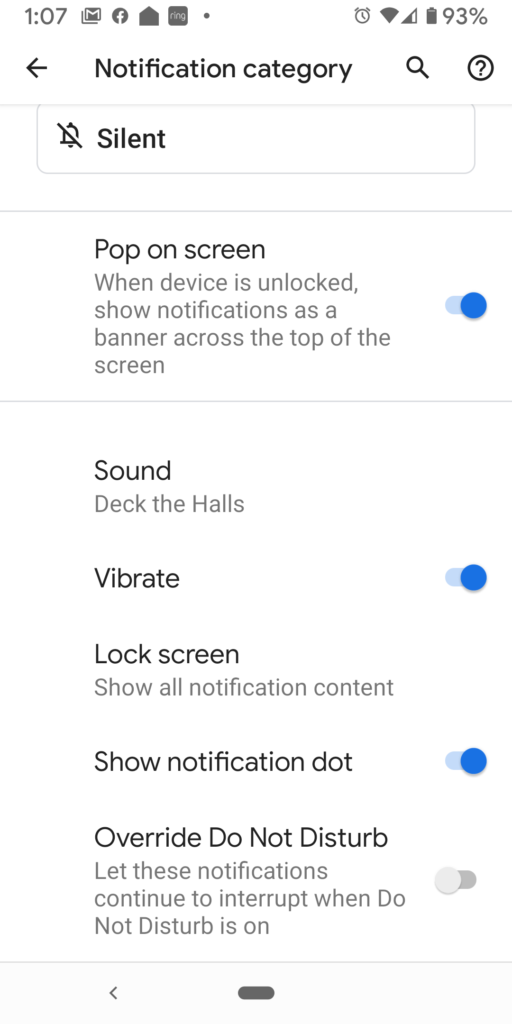Descriptive Caption:
---
The image appears to be a screenshot of a smartphone settings screen with various notification options. The top of the screen displays a status bar showing icons for Gmail, Facebook, a house, and Ring.com, along with indicators for full WiFi signal, 93% battery, and a left arrow for navigation.

Below the status bar, the main settings screen lists different categories related to notifications. These include a penetration category and options highlighted with icons such as circles and question marks. A specific setting for "Pop on screen when device is unlocked" is visible, indicating the option to show notifications when the device is active. 

A banner spans across the top of this section, containing a blue toggle switch for enabling notifications. Beneath the banner, there's a divider line separating the different settings.

Further options include sound settings and decal options, followed by a vibrate toggle switch. The lock screen settings allow users to "Show all notification content" and feature a blue toggle for "Show notification dot." Another blue toggle option, labeled "Override Do Not Disturb," permits certain notifications to bypass the Do Not Disturb mode.

The interface includes additional divider lines and a grey oval button for navigation. The background of the screen is very white, contrasting with the various icons and text. Each section provides users with detailed control over their device's notification behavior.